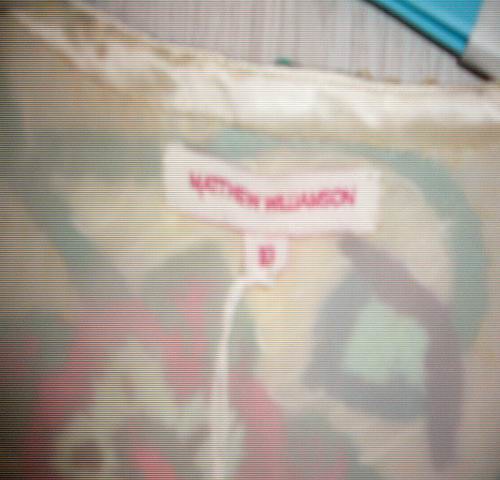A close-up image captures a delicate garment, seemingly a woman’s piece, turned inside out. The fabric is a sheer, cream-colored material complemented by a satin waistband. Prominently featured is a white tag with magenta-pink lettering, likely indicating the brand "Matthew Williamson." Although somewhat blurred, the tag also appears to display a size, potentially a size 10, though it's indistinct. The garment itself showcases a captivating design in purple, turquoise, magenta, and white hues. In the background, a turquoise blue metal pole capped with white hints at a laundry apparatus, contributing to the scene's domestic atmosphere.